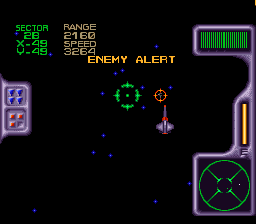The image is a small, rectangular screenshot from a video game, with dimensions that are slightly wider than it is tall. The screen background is predominantly black, suggesting a deep space setting. In the upper central portion of the screen, just above the midpoint, there's a conspicuous green target-like icon. This green icon features a bright green dot at its center and is composed of several semi-circles positioned at the top, bottom, left, and right, which are not fully connected, creating a radar-like appearance.

To the right of this green icon, there's a much smaller version of a similar icon, which is red in color. Below this red target, there is a top-down view of a digital spaceship, advancing upwards. The spaceship is primarily lavender in color with some red accents, featuring two wings and a long, pointed nose.

Above the green icon, the text "ENEMY ALERT" is prominently displayed in all capital letters with a vivid orange color. To the upper left side of this text, two sections of information are presented. The left section, outlined in green text, reads "SECTOR," followed by "28," "X-49," and "V-49" in descending order. The right section, enclosed in a light brown box, contains the text "RANGE" followed by "2160," "SPEED," and "3264," all in capital letters.

The right side of the image is predominantly obscured by a shape outlined in lavender blue, covering a substantial portion of the area. Located at the bottom-right is another green circle with four lines extending inward from its circumference, resembling a secondary target indicator. This indicator is outlined in lavender, matching other visual elements on the screen. Thin horizontal and vertical green lines fill this area, creating a dense grid-like pattern, which contributes to the overall digital, high-tech aesthetic of the image.